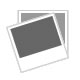This photograph captures a detailed close-up of an old, worn radio tuner clutched by a pale, older-looking hand with a ring on one finger, suggesting it belongs to an older male. The radio features a green plastic casing in a shade reminiscent of avocado or lime, with two prominent, silver knobs— each with a black interior. The top knob, labeled "tuning," adjusts frequencies ranging from 5.4 to 16 megawatts (MW) and displays a notation of "times 100 kilohertz." The lower knob, marked "volume," has a scale from 1 to 10 and includes an "off" option. Both knobs rest against a black rectangular background. The hand's aged appearance contrasts with the vibrant green of the radio, emphasizing its vintage charm and the probable long-term use of the device.